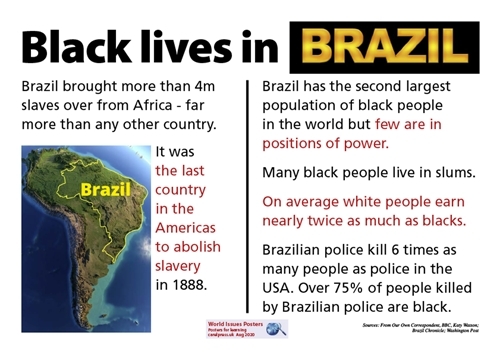This image depicts a visually striking news article about racial issues in Brazil, set against a white background. The prominent headline reads "Black Lives in Brazil," with the word "Brazil" highlighted in yellow letters within a black box. The article emphasizes that Brazil imported over 4 million slaves from Africa—more than any other country—and was the last nation in the Americas to abolish slavery in 1888.

A visual representation of the country of Brazil is included, with the map outlined in yellow on a blue background. The right side of the page features critical statistics: Brazil has the second-largest population of Black people in the world, yet few hold positions of power, and many reside in slums. The article highlights the economic disparity where, on average, white Brazilians earn nearly twice as much as their Black counterparts. Furthermore, it notes that Brazilian police have a much higher rate of killings compared to the USA, with over seventy-five percent of those killed being Black.

At the very bottom, there is a small purple box containing some additional writing, and a blue circle with a line through it. The sources for the information presented are listed in black at the end of the article.